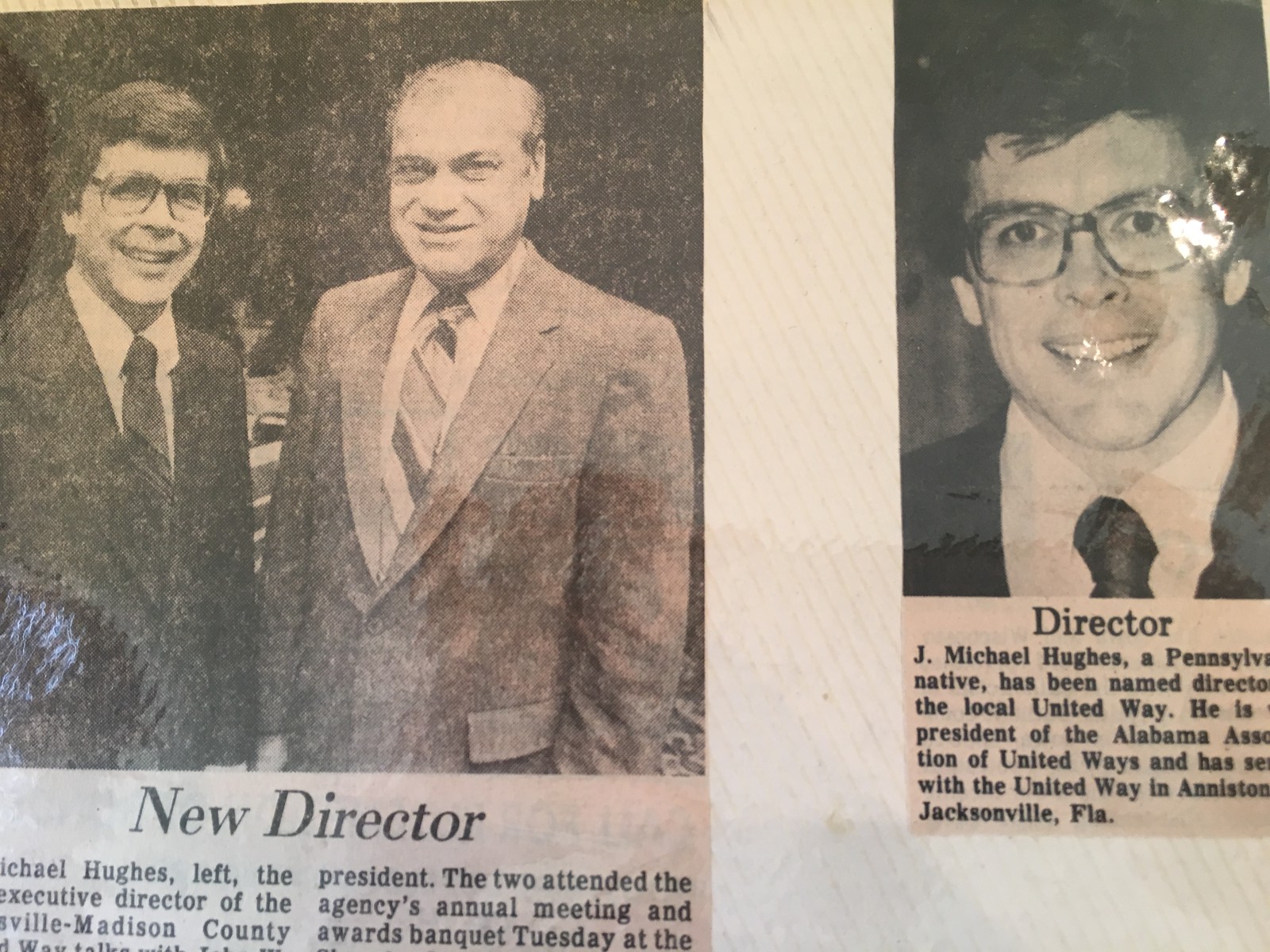The image displays two adjacent newspaper clippings, likely from the 1960s or 70s, positioned side-by-side on what appears to be a scrapbook page. Both clippings feature portraits of men in suits. On the left clipping, two men are standing side-by-side, smiling directly at the camera. The younger man on the left, likely in his 30s, wears glasses and a suit with a tie, while the older man on the right, probably in his 50s, is balding and also dressed in a suit and tie. The accompanying headline reads "New Director," with text partially obscured, noting "Michael Hughes left the president" and mentioning attendance at an annual meeting and awards banquet in Madison County. 

The right clipping features a close-up of a man identified as J. Michael Hughes, a Pennsylvania native, named as the new Director of the United Way. He is also President of the Alabama Association of United Ways and has served with United Way in Anniston, Jacksonville, Florida. He sports glasses and a suit, smiling warmly at the camera. The predominant colors in the image are black, white, varied shades of gray, and hints of off-red, all contributing to the vintage newspaper aesthetics.